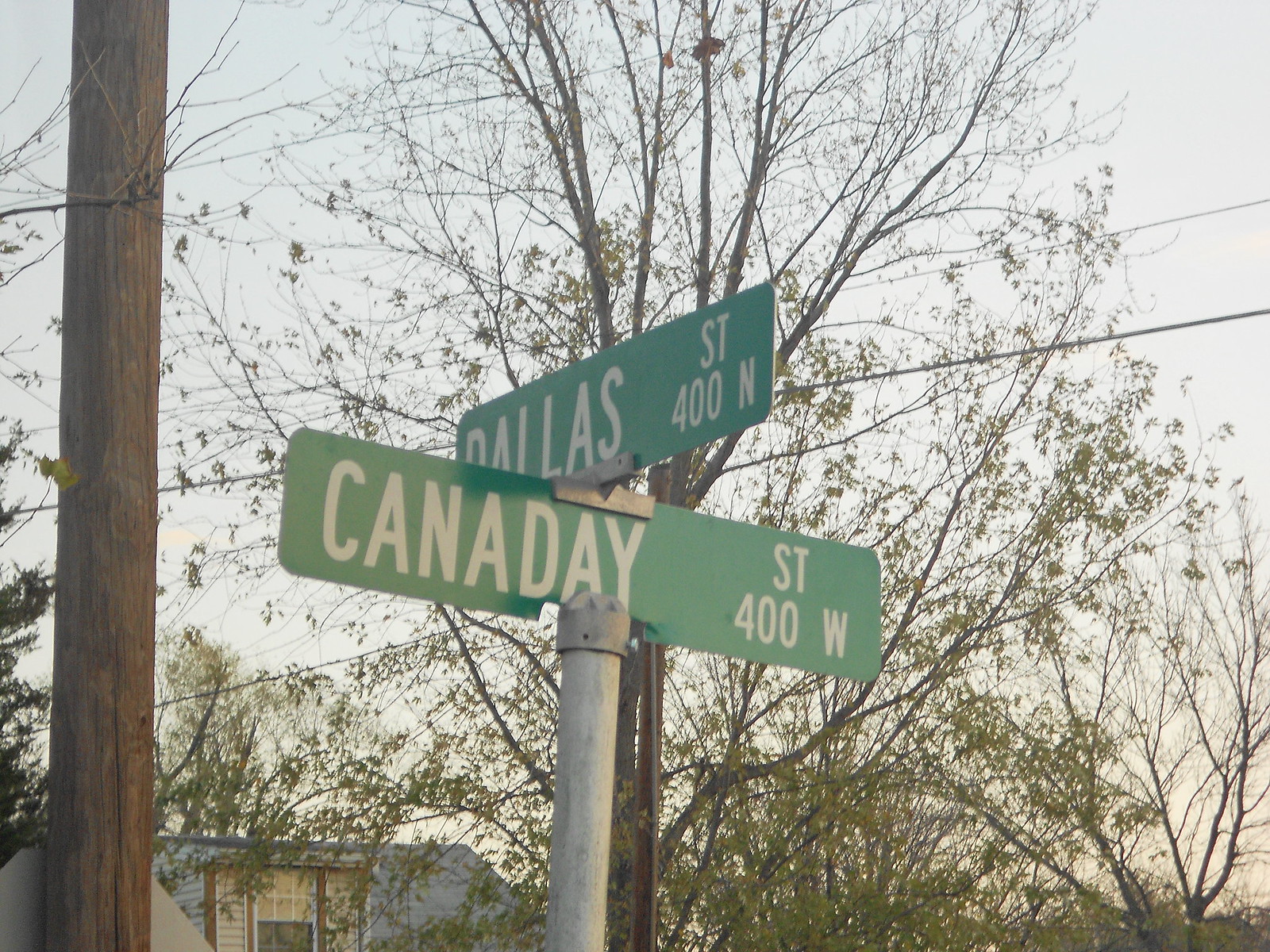This photograph captures an outdoor scene with a distinctive street sign at its center. The sign, mounted on a silver metal pole, displays two horizontal green rectangles with white lettering. The lower sign clearly reads "Canaday Street 400 West," while the upper sign, slightly cut off, shows "Dallas Street 400 North." The background features a large, mostly dormant tree, its myriad branches stretching across the scene with only a few budding leaves, suggesting early spring. The sky above is a bluish-gray, perhaps hinting at dusk, with a hint of yellow glow near the horizon. To the left edge of the image, a thick wooden telephone pole runs vertically. Also visible in the background is the roof of a house with a gray exterior and a window jutting out from the second floor. Another detail in the lower left corner is a small trailer, adding to the image's composed yet rustic feel.